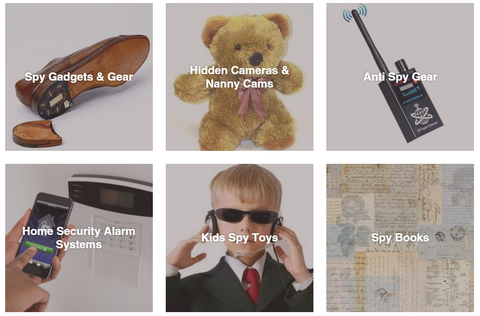The image is a horizontally aligned rectangular grid composed of six equal squares, each bordered by white stripes. Arranged in two rows of three, each square showcases a different category in white text across the center, accompanied by a representative image. 

The top left square features a shoe with its heel removed, labeled "Spy Gadgets and Gear." The top center square displays a brown teddy bear under the title "Hidden Cameras and Nanny Cams." To the right, the top right square depicts a handheld device with an antenna, marked "Anti-Spy Gear."

In the bottom row, the lower left square shows a person's hand holding a cell phone beside an alarm box, labeled "Home Security Alarm Systems." The bottom center square features a young boy in a suit, tie, sunglasses, and headset, titled "Kids' Spy Toys." The final square, in the lower right, presents scattered pages of text, under the heading "Spy Books."